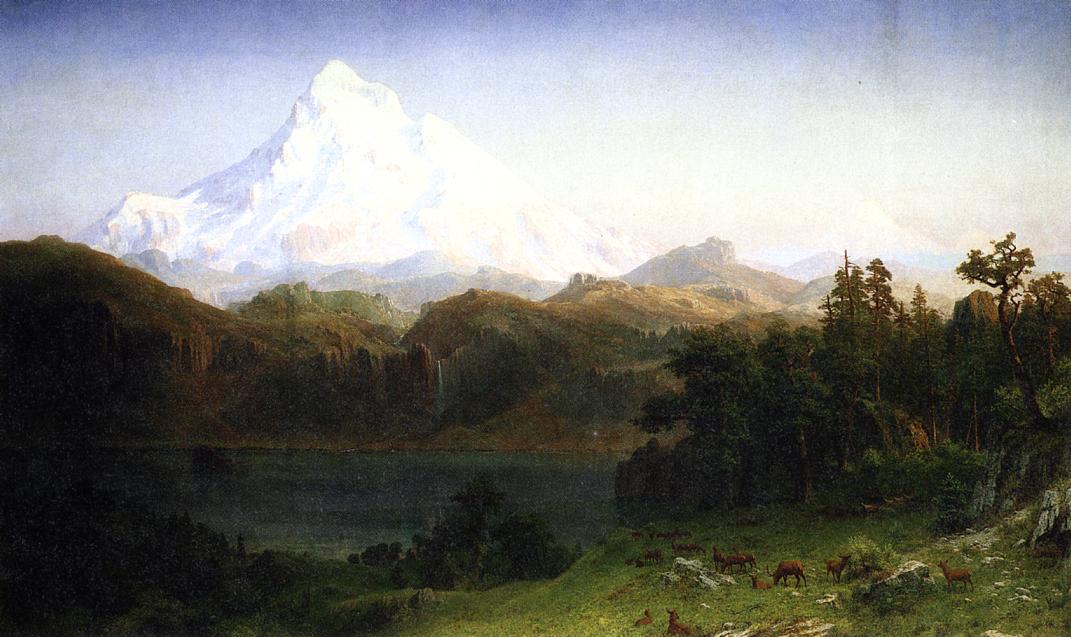This is a wide, rectangular painting of a stunning landscape, probably inspired by the Matterhorn due to its distinct pointed, snow-capped peak. The sky at the top of the painting is a very pale, grayish-blue, and features a very tall, white, snowy mountain on the left that broadens into shorter mountainous terrain to the right. Below this majestic peak, a range of dark green and brown hills extends across the image, tallest and darkest on the left before dipping and rising again, then fading into the right. A very dark, bluish-green body of water rests at the base of these hills, embraced on the right by a thick forest of tall, dark green trees. The foreground of this picturesque scene features a bright, green, grassy area with several brown, four-legged animals that resemble goats or deer grazing. Overall, the painting transitions from the light, airy sky to the darker, lush, pastoral setting below, capturing the serene and dramatic elements of this natural landscape.